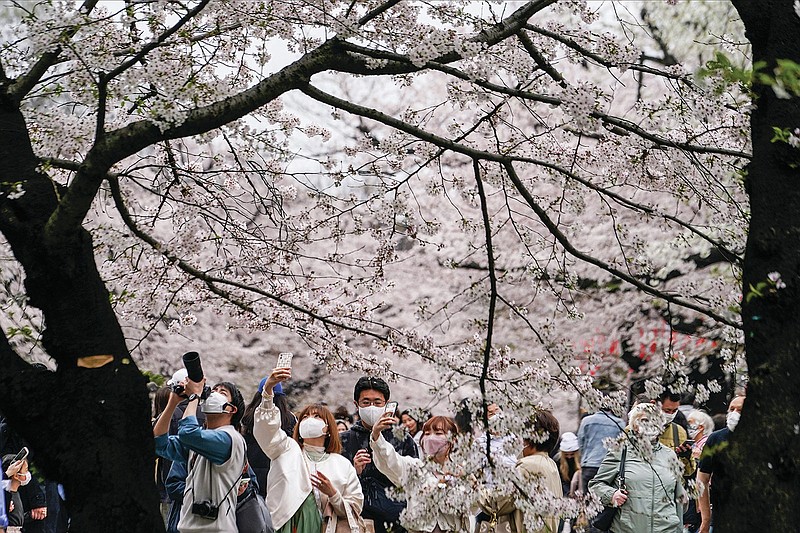In a sunlit park during the COVID-19 pandemic, a large group of young Asian adults, all wearing white respiratory masks and dressed in sweaters or life jackets, gather closely together beneath the vibrant canopies of fruit trees. The scene is suffused with a bright, white tint, giving it an almost ethereal quality as sunlight filters through the dense, willowy branches laden with striking white blossoms. The image captures the upper expanse of the trees, their dark, rugged trunks grounding the delicate, sprawling branches above. At the bottom of the picture, the crowd holds up cameras and cell phones, intently capturing the beauty of the flowering trees. The composition highlights the contrast between the lively, natural canopy and the multitude of masked faces, creating a poignant image of communal appreciation for nature amidst a time of global health crisis.